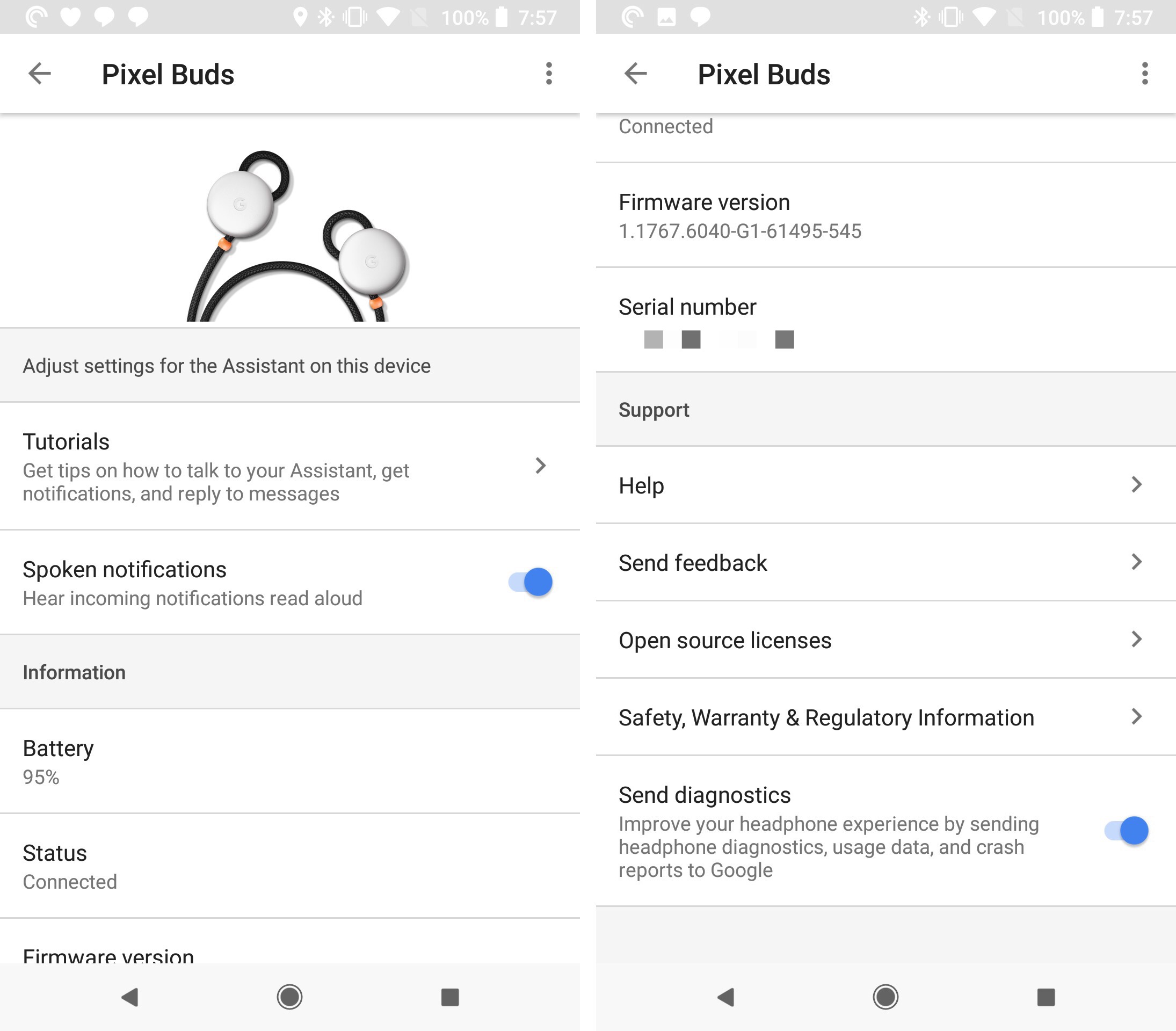**Detailed Caption for the Screenshot of a Cell Phone Display**

**Left Screenshot:**

- **Top Bar:**
  - A horizontal gray bar with several icons:
    - A three-quarter closed circle icon on the left.
    - A white heart icon.
    - Two messaging icons.
    - A location icon.
    - A Bluetooth icon.
    - A silent mode icon.
    - An internet access icon.
    - The text "100%" in white.
    - A full battery icon in white.
    - The time "7:57" on the far right.
    
- **Header:**
  - Background: White.
  - A left-facing arrow on the left.
  - The text "Pixel Buds" in black, aligned to the right of the arrow.
  - A more options/settings icon on the far right.

- **Main Content:**
  - An image of Pixel Buds is displayed in the middle.
  - A gray bar with the text "Adjust settings for the assistant on this device" in gray.
  
- **Options:**
  - "Tutorials" in black letters.
  - Underneath: "Get tips on how to talk to your assistant, get notifications, reply to messages" in gray, with a right-facing arrow to the right.
  
- **Notification Settings:**
  - Title: "Spoken notifications" in black.
  - Description: "Hear incoming notifications read aloud" in gray, with a toggle switch on the right (turned on).
  
- **Information Section:**
  - Title: "Information."
  - Subtitle: "Battery" in black, followed by "95%" in gray.
  - Subtitle: "Status" in black, followed by "Connected" in gray.
  - At the bottom: "Firmware version" in black, partially cut off in the screenshot.
  
- **Bottom Navigation:**
  - A left-facing arrow.
  - A gray circle.
  - A gray square to the right of the circle.

**Right Screenshot:**

- **Top Bar:**
  - A horizontal gray bar with several icons:
    - A three-quarter closed circle on the left.
    - A picture button.
    - A messenger icon.
    - A Bluetooth icon.
    - A silent mode icon.
    - An internet access icon.
    - The text "100%" in white.
    - A full battery icon in white.
    - The time "7:57" on the far right.
    
- **Header:**
  - A left-facing arrow on the left.
  - The text "Pixel Buds" in bold black letters, aligned to the right of the arrow.
  - A more options/settings icon on the far right.

- **Status Information:**
  - "Connected" in gray.
  - "Firmware version" in black, followed by "1.1767.6040-G1-61495-545" in gray.

- **Serial Number Section:**
  - Subtitle: "Serial number" in black.
  - Next to an image of a small gray square, a black square, and a dark gray square with small spacing between them.

- **Support Section:**
  - A highlighted rectangular area in gray with the text "Supports" in black.
  - Below this: "Help" in black with a right-facing arrow on the right.
  - Next: "Send feedback" in black with a gray right-facing arrow on the right.

- **Legal Information:**
  - "Open source licenses" in black with a gray right-facing arrow on the right.
  - "Safety warranty and regulatory information" in black with a right-facing arrow on the right.
  
- **Diagnostics Section:**
  - Title: "Send diagnostics" in black.
  - Description: "Improve your headphone experience by sending headphone diagnostics usage data and crash reports to Google" in gray, with a toggle switch on the right (turned on).